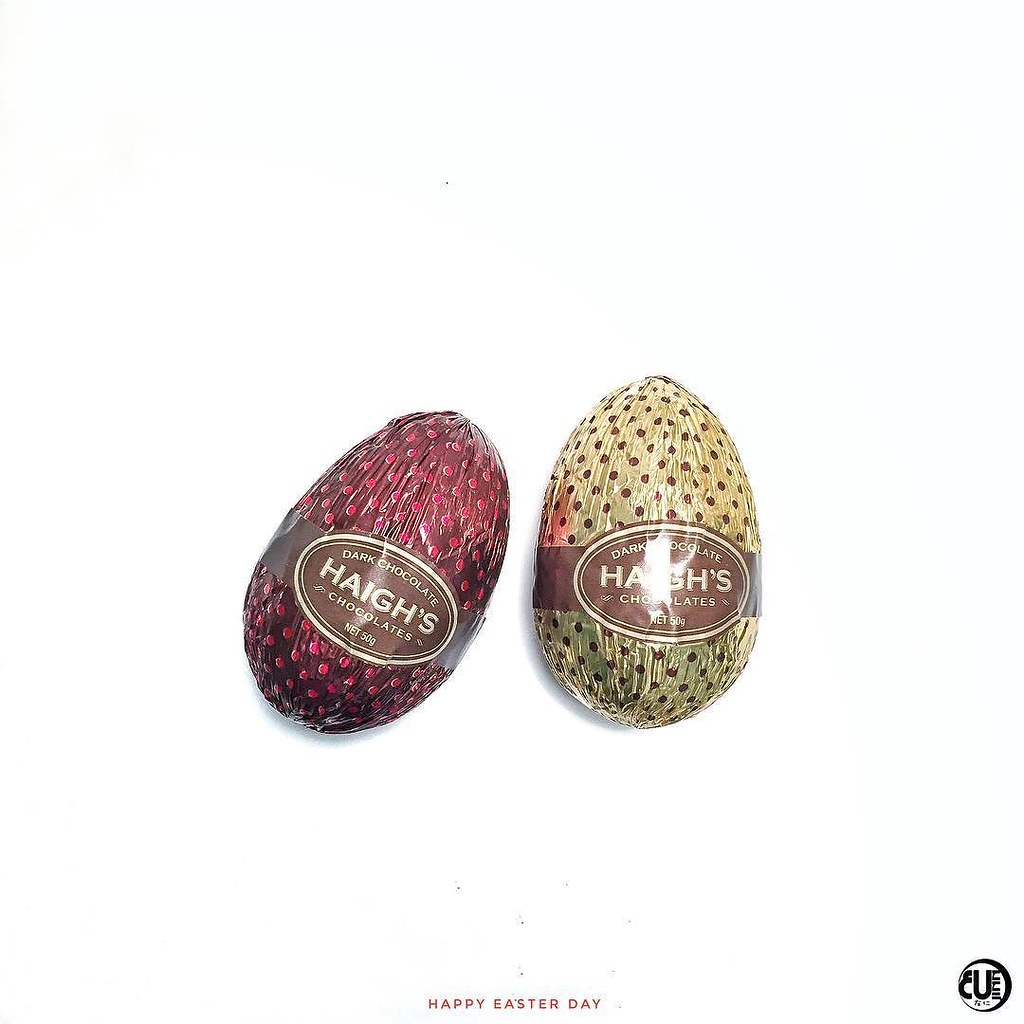The image features two foil-wrapped chocolate Easter eggs set against a stark white background. The egg on the left is wrapped in a dark purple foil with pink polka dots, while the egg on the right is wrapped in a golden foil adorned with little brown dots. Both eggs have identical brown horizontal bands in the middle, displaying the text "Haigh's Chocolates" along with the weight of "50 grams." Additionally, they are labeled "Dark Chocolate." Below this, the text "Happy Easter Day" is written in a brownish-red font. Positioned in the lower right corner is a black and white logo. No people are present in the image.